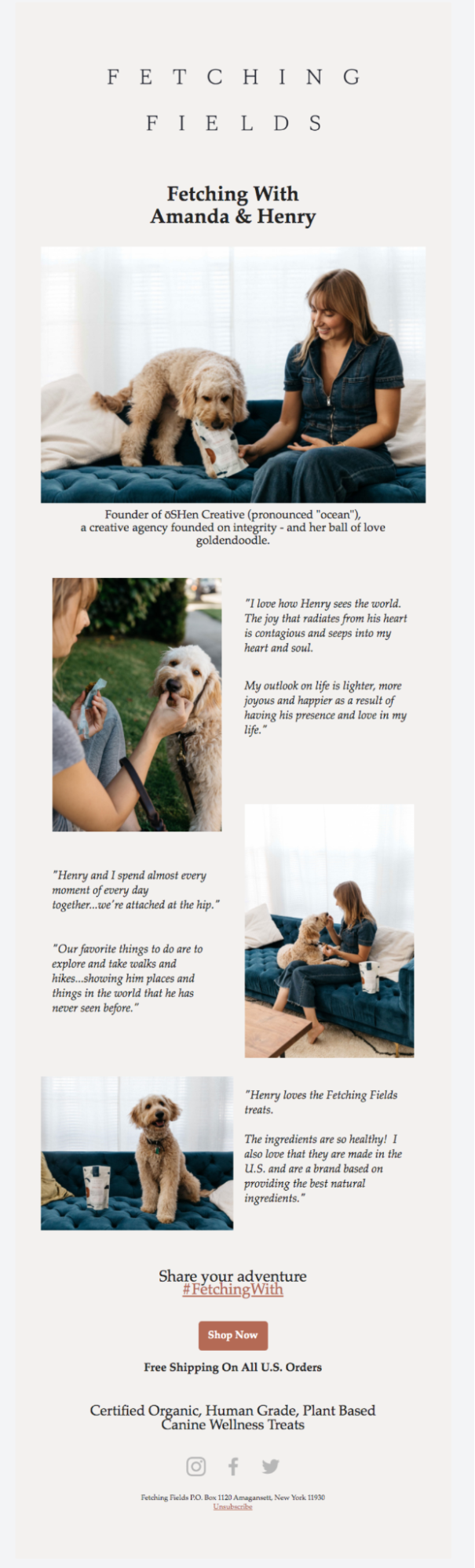In the upper center of this image, the text "Fetching Fields" is prominently displayed. A few inches below, it reads, "Fetching with Amanda and Henry." The main image on the right features a woman with light brown hair and bangs, seated on a dark green surface. She is dressed in a dark green, short-sleeved outfit with buttons. In her hand, she holds a bag of food, which she offers to a light brown dog standing on the same green cushion. The dog's mouth is near the package, indicating its interest.

The second image, positioned to the left, shows the same woman sitting outside on the grass. She is wearing a gray short-sleeved shirt and holds a blue item in her left hand. In her right hand, she is feeding the same light tan-colored dog.

Below this, the picture on the right provides another view of the woman and the dog on the green couch. The final image on the left captures the dog alone on the green couch surface. Underneath, in orange text, it says, "Share your adventure, #FetchingWith."